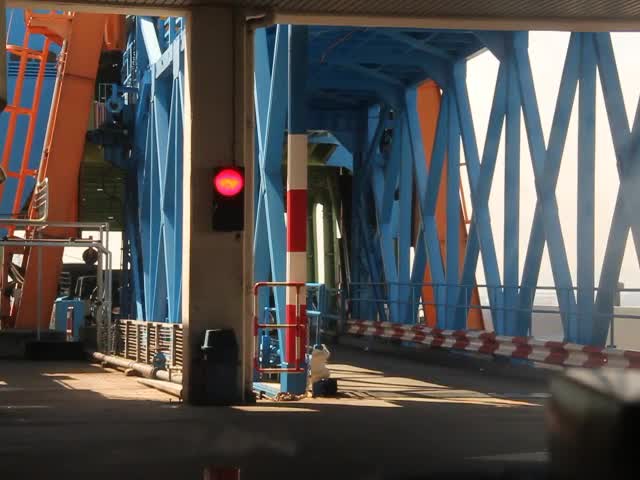An interior view of a bridge showcases vibrant structural elements and functional design. The bridge features sturdy blue metal beams on its exterior, while the top structure is painted in a striking orange hue. The design includes a series of metal diamond patterns that provide support and add visual interest. On either side of the bridge, there are handrails that run along the bottom edge, ensuring safety for pedestrians.

The floor of the bridge is constructed from durable concrete, offering a solid walking surface. As one enters the bridge, a red and white pole-like object is mounted to the ground on the left side, possibly serving as a marker or a boundary indicator. In the distance, to the far left, there is an individual handling a couple of suitcases, suggesting that the bridge connects to a transit or travel facility. The suitcases, along with the person handling them, add a touch of human activity to the otherwise industrial scene.